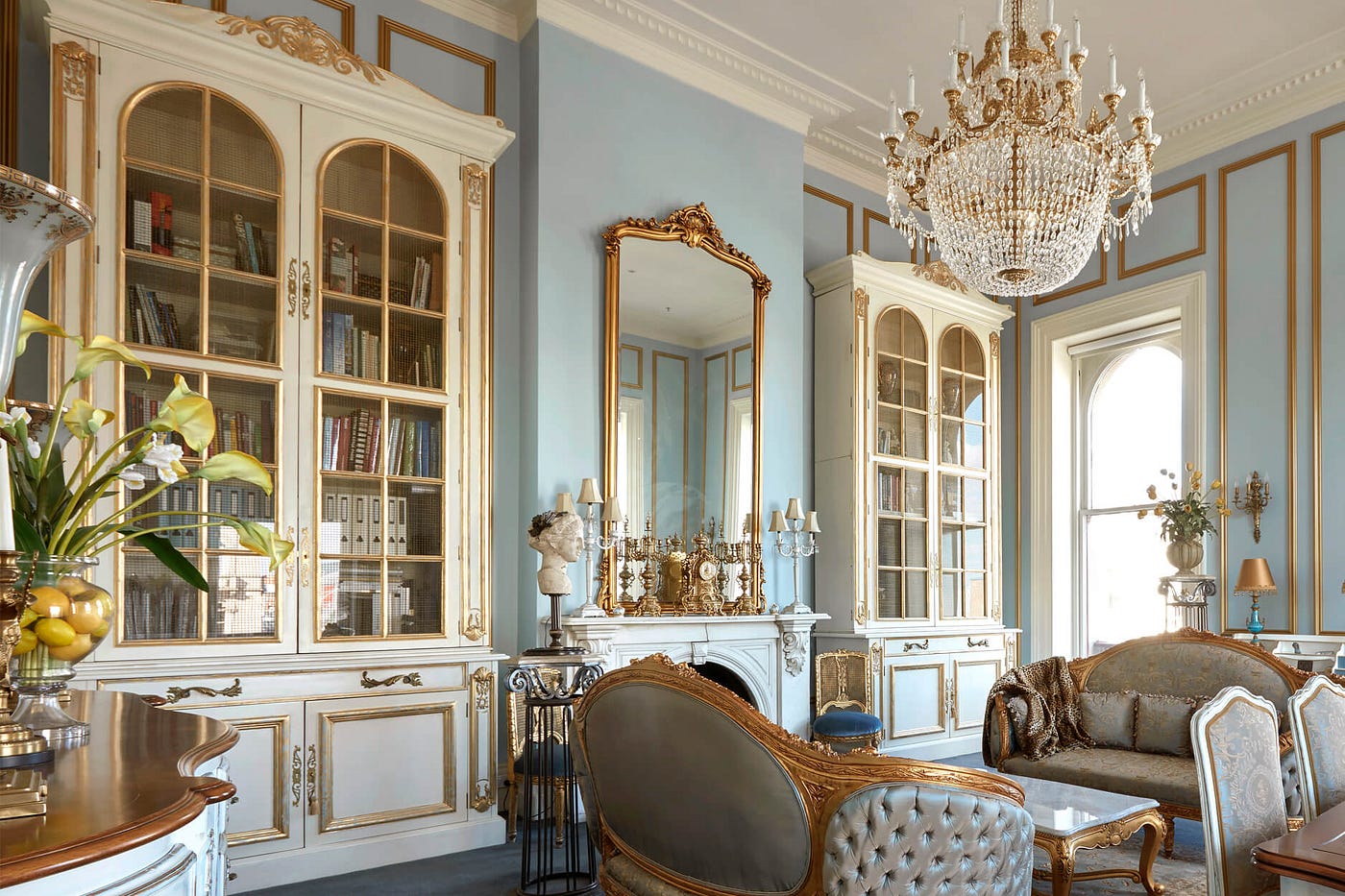This photograph captures the interior of an opulently decorated, sunlit room reminiscent of palace interiors. The light blue walls and white ceiling create a bright and airy atmosphere, complemented by the sunlight streaming in. A large, white bookcase with ornate gold decorations stands on the left, extending up to the ceiling and filled with books. A central feature of the room is an elegant mantelpiece with a grand mirror above it, both featuring intricate gold detailing. This mirror and fireplace are positioned prominently on the room’s left side. An additional matching bookshelf is visible towards the right. On the floor, an assortment of ornate furniture is arranged, including couches, chairs, and a table, all showcasing gold-trimmed embellishments. A medium gray rug lies underneath these furnishings, tying the room together. Completing the lavish setting is a magnificent chandelier with gold accents, hanging from the white ceiling.